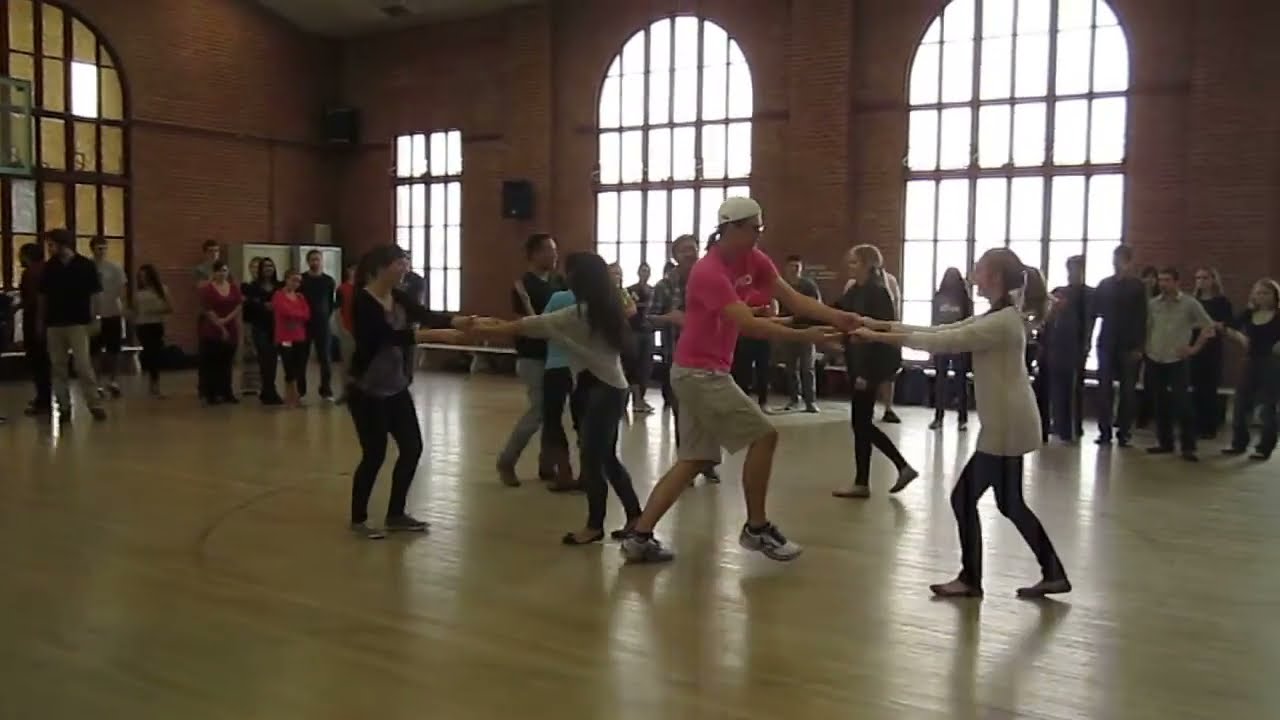The photograph depicts a lively scene inside a dance studio, featuring a light brown, shiny wooden floor. The studio's red brick walls are accentuated by three large arched windows, with two along the outer walls letting in ample natural light, and the third, situated inside, possibly opening to a hallway. Additionally, there's a rectangular window adding further light to the space. The ceiling appears white, giving the room an airy feel.

In the center of the room, several couples are actively engaged in dance, flanked by a crowd observing from the perimeter. The dancers and onlookers are diverse in appearance: a man in a black shirt, gray undershirt, and black pants dances with a woman in a white shirt and jeans. Another male dancer wears a dark shirt and white pants, partnered with a woman in a blue shirt and dark pants. At the forefront, a man in a pink shirt, khaki shorts, and a white hat, possibly with glasses, dances with a woman in a white shirt and dark pants. Around them, spectators are mostly dressed in darker clothing, with a notable couple on the left in dark clothing and khaki pants, and another pair in whitish shirts and dark pants. 

The background is rich with details such as ballet poles, signs, speakers, and a variety of colors, including pink, beige, white, black, tan, brown, cream, cyan, blue, purple, navy, and orange. The observers create a sort of square around the dancers, adding to the structured yet lively atmosphere of what appears to be a dance class or possibly a rehearsal.